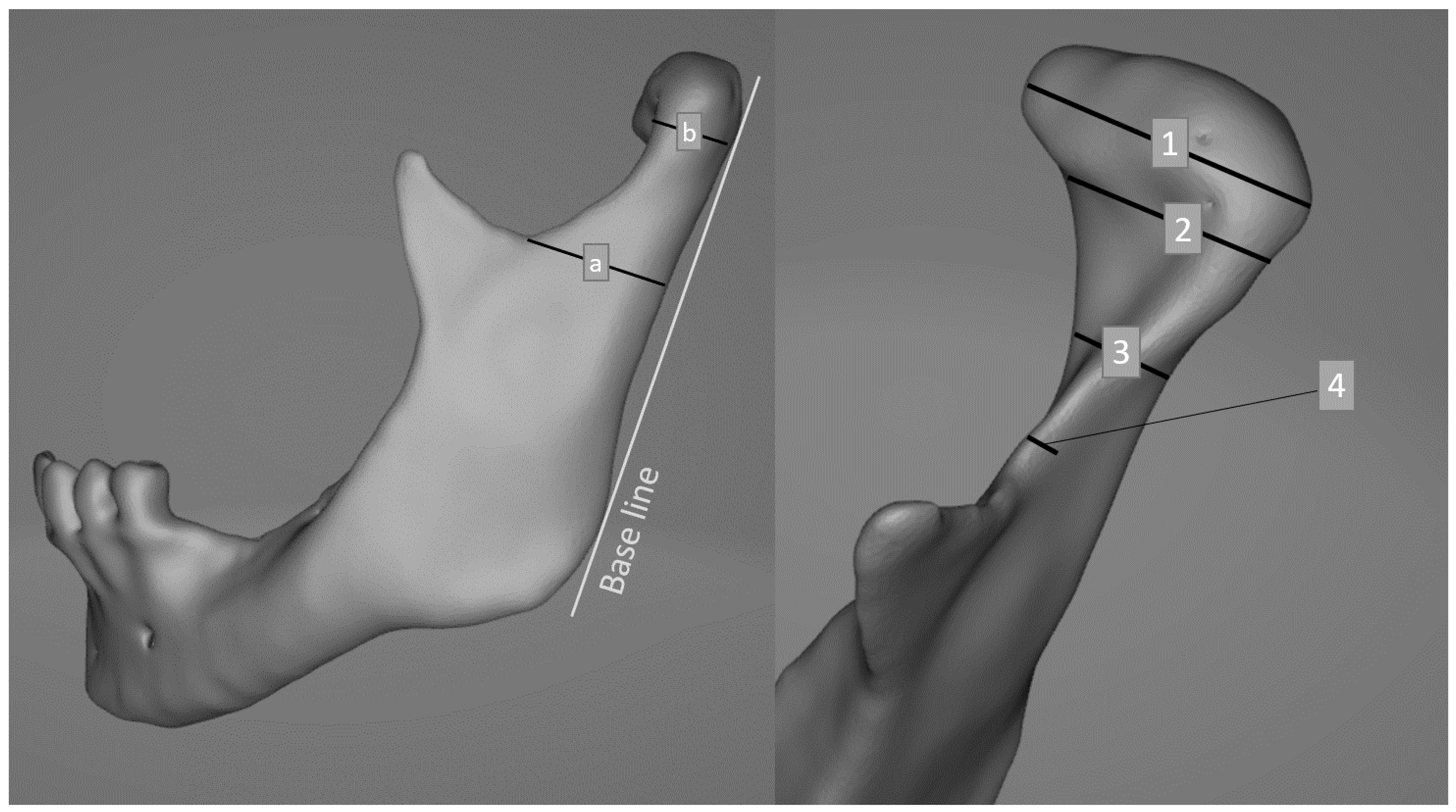This black-and-white computer-generated 3D rendering features two grayscale images of a human jaw. On the left, the image depicts the left half of a bottom jawbone with teeth, characterized by a baseline that separates the foot from the protruding toes. The diagram includes labels such as 'A' and 'B' and a white line running the length of the jaw. On the right, a side profile of the jawbone is shown from a different angle, possibly the inner side, with numbered sections 1 through 4 and black lines indicating various anatomical points. The overall composition suggests a detailed medical rendering likely used for anatomical study or the creation of 3D-printed medical models.